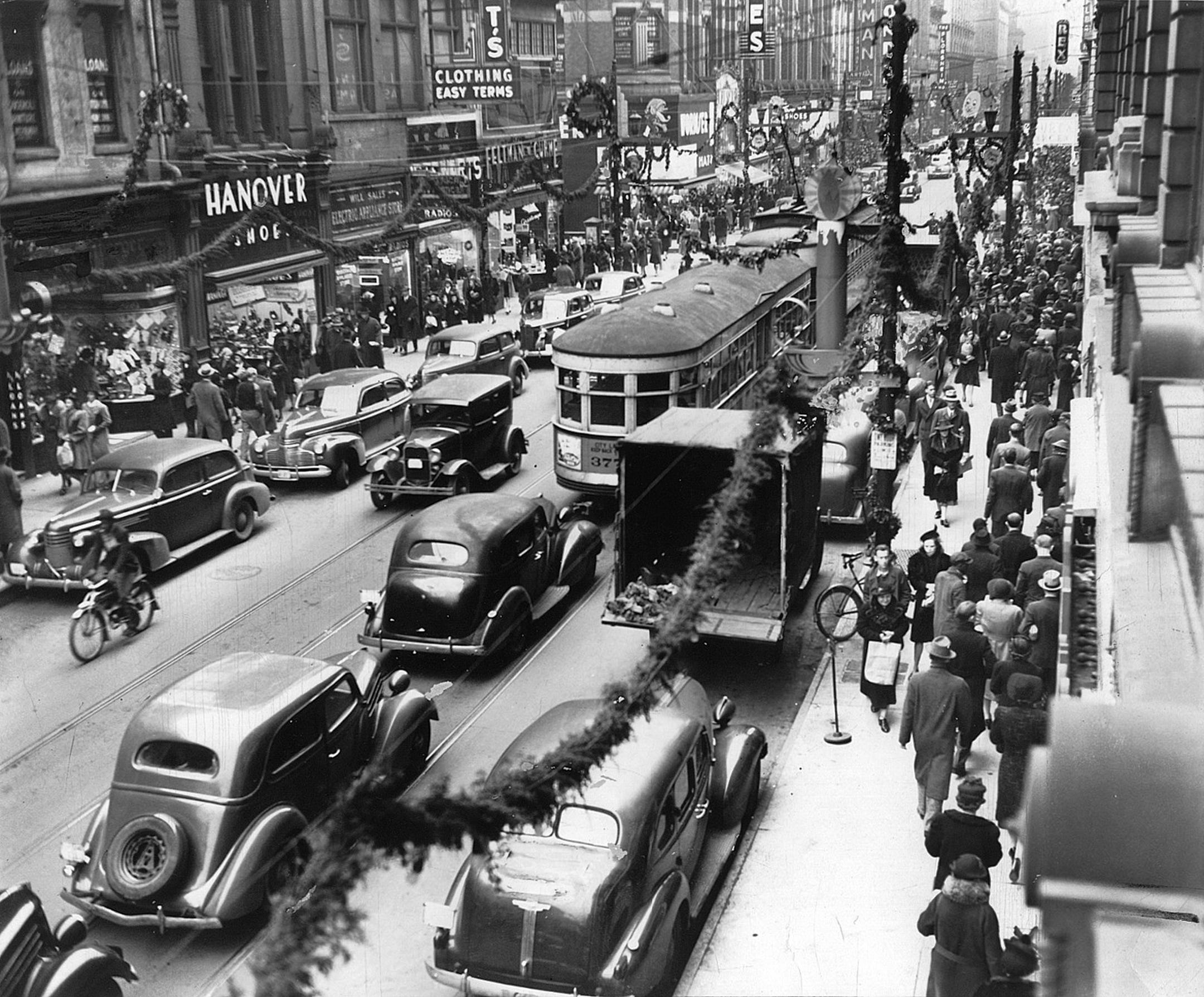This vintage black-and-white photograph, likely taken from an elevated viewpoint like a window or balcony in the 1930s, presents a bustling city street during Christmastime. The sidewalks are densely packed with people, all dressed in coats appropriate for the winter season. The street itself is lively, featuring an array of vehicles including old-school Model T-type cars, bicycles, and an electric trolley or tram. The festive atmosphere is vividly captured through the decorations, with garlands strung along the power lines and Christmas wreaths adorning streetlamps and storefronts.

The storefronts provide a snapshot of the era's commercial activity, with visible signs for Hanover Shoes, TNS Clothing, and a Rexall Drugstore among others. The image is rich in historical detail, showcasing a time when downtown retail districts thrived with shoppers getting into the Christmas spirit. The visual composition, with its contrasts in lighting and busy street scene, makes this a classic representation of urban life in the 1930s, imbued with a sense of nostalgia for a bygone era.